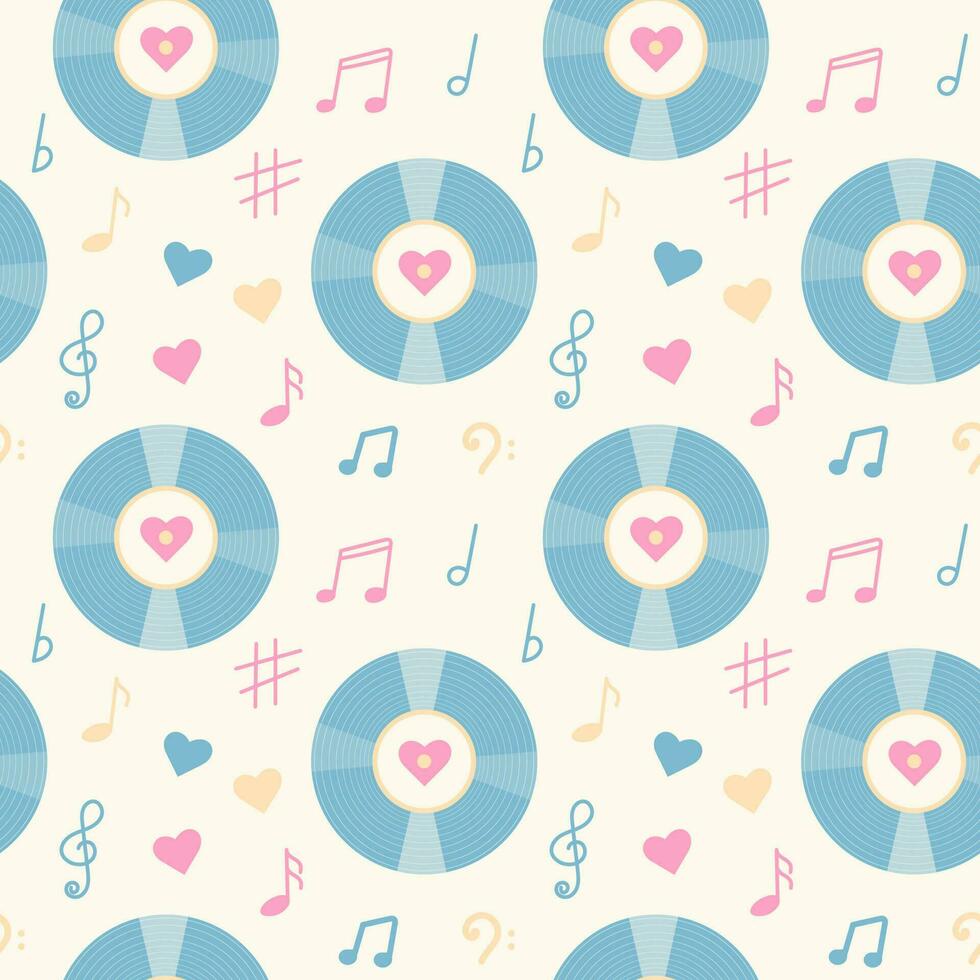The image depicts a square section of wallpaper or wrapping paper, designed with a vibrant 1950s motif. The background is a faded, off-white hue, giving it a vintage feel. Central to the design are repeating patterns of large blue records, reminiscent of 45 RPM vinyl discs, each featuring a pink heart with a small golden dot at its center. Scattered in between these records are various music symbols, including clefs, notes, and symbols, in pastel shades of pink, blue, and yellow. Additionally, small hearts in matching colors are interspersed throughout the pattern, adding to the musical and retro aesthetic. The pattern is meticulously organized, with full records flanked by partial ones along the edges, creating a seamless, continuous design that recalls classic wallpaper styles.